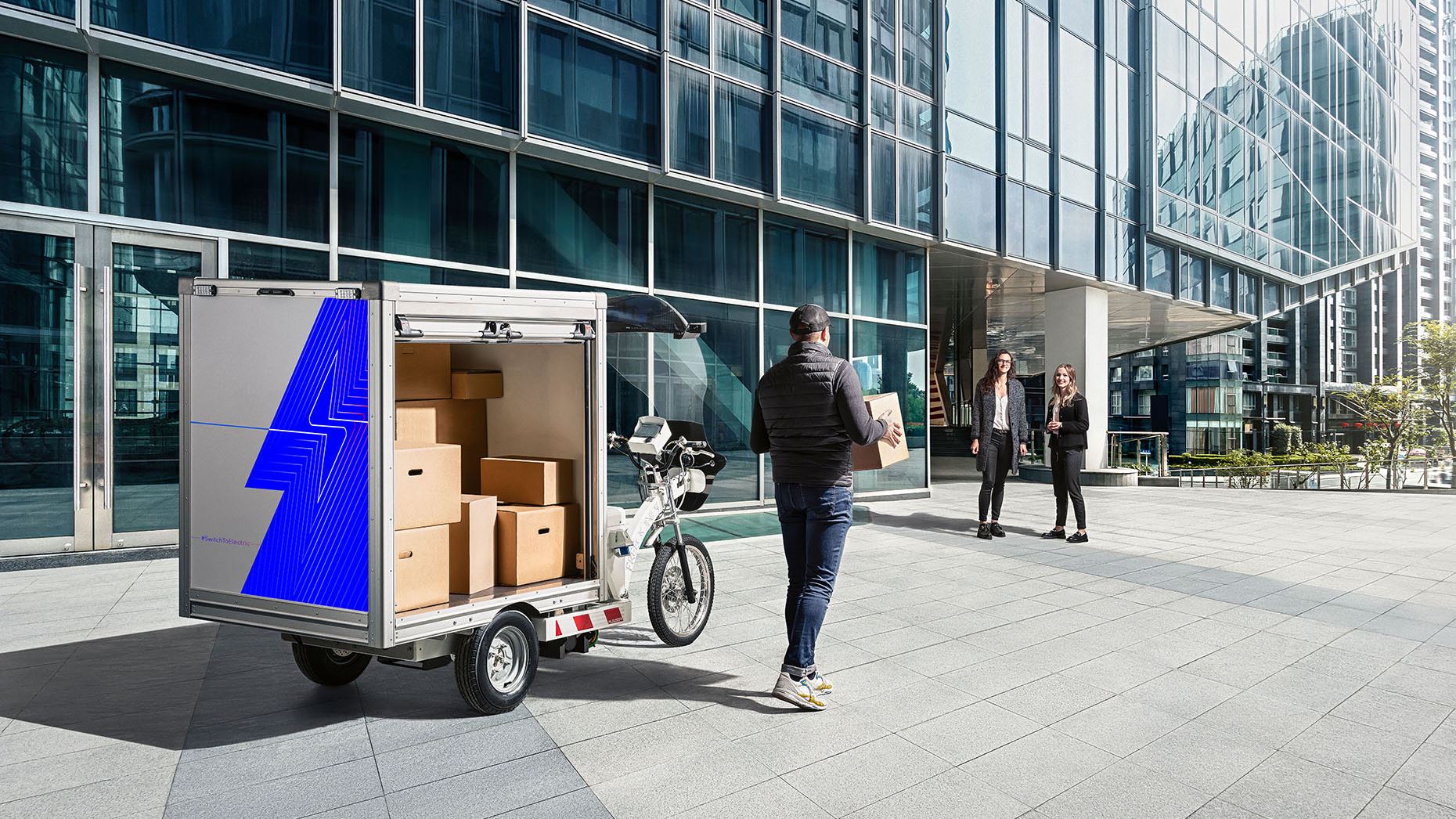In this full-color, horizontally rectangular photograph taken outdoors in daylight, the scene is set in a large city in front of a multi-story glass building. The reflections on the glass reveal at least one other multi-story building nearby. The foreground showcases a patterned pavement of white and gray blocks. Central to the image, a man dressed in navy blue jeans, a dark gray top, and a hat is walking towards two young women who are in business casual attire. The man clutches a cardboard box, his face obscured. Positioned to his left is a peculiar delivery vehicle, a tricycle motorcycle with a large storage container bearing a royal blue lightning bolt emblem. This container is packed with more light brown cardboard boxes, indicating his role as a delivery person. The glass building's windows exhibit a blue tint, while the overall palette of the photograph includes blues, grays, browns, blacks, and whites, capturing the urban atmosphere and the routine of package delivery.